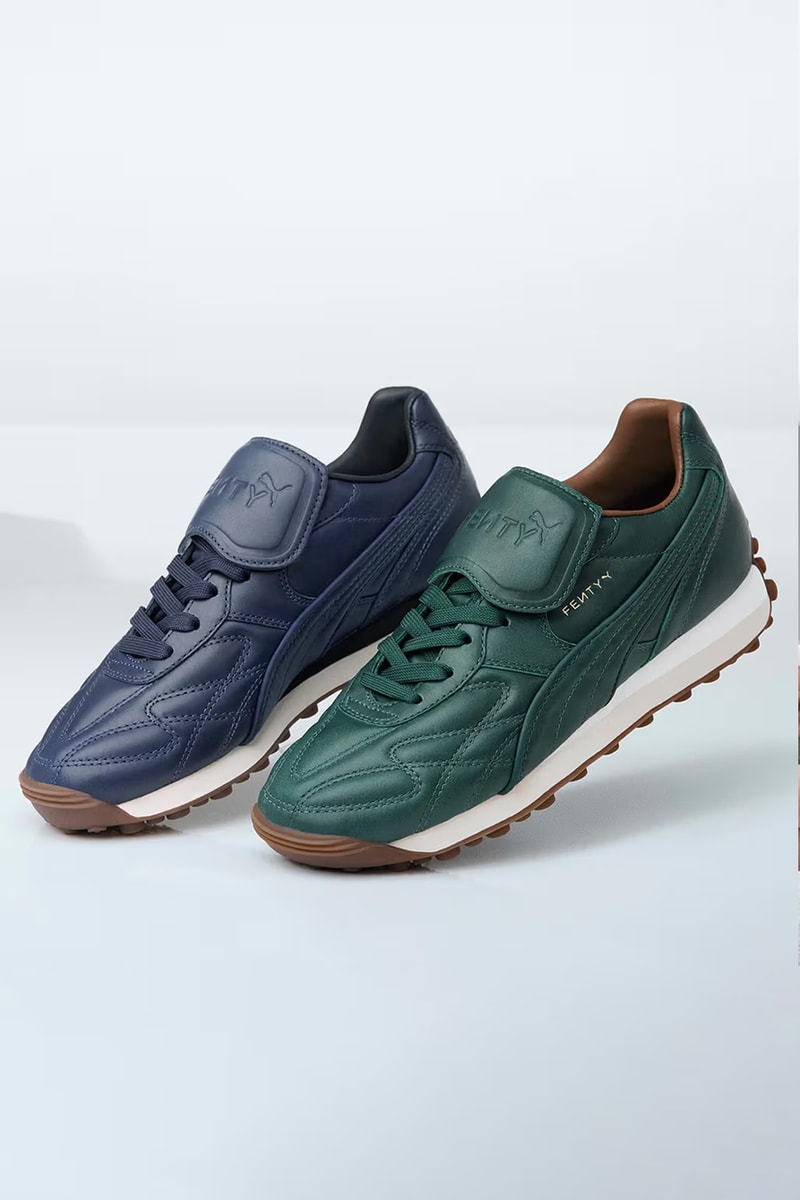This image features a pair of sneakers set against a gray background with light shadowing. The sneakers, made by the brand Venti, are presented in two different color schemes but share a common design. The left shoe is predominantly dark blue with a brown toe guard, while the right shoe is mainly dark green, also with a brown toe shield and brown interior heel. Both shoes feature a notable white stripe around their base and brown soles with a ripply edge at the bottom.

The shoes are equipped with both laces and a prominent velcro strap across the top, partially covering the bow-tied laces. The left shoe has a Venti branding on the velcro strap, while the right shoe displays the brand's name, 'FENTYY'—notably with a backward 'N'—in white text under the strap on the side. The interior of the left shoe is black, and the right shoe's interior is brown. Positioned in the center of the image, the heels of the shoes are raised, pointing slightly downward towards the left, creating an angled view that showcases their unique and contrasting color patterns.